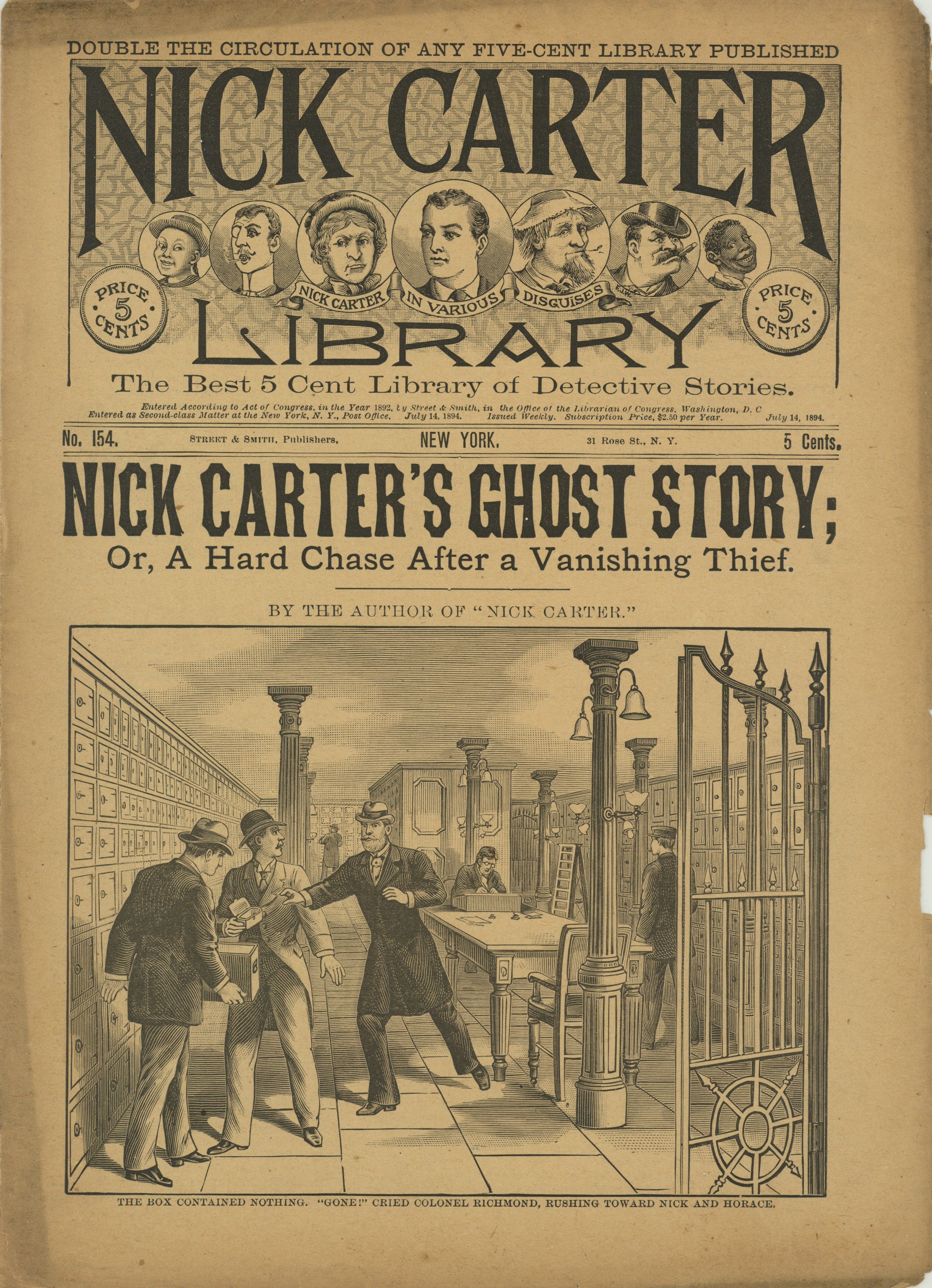An old newspaper cutout, primarily in shades of brown and black, boasts "Double the circulation of any five-cent library published." It features the renowned "Nick Carter Library," hailed as the best five-cent library for detective stories. Prominently displayed is an advertisement for "Nick Carter's Ghost Story, or A Hard Chase After a Vanishing Thief" by the author of Nick Carter. In the scene depicted, a man dressed as a private detective, complete with a long trench coat and bowler hat, reaches out towards two men in suits and hats as they examine a box inside a bank vault filled with lockers. In the background, a man works at a table while another, possibly security, patrols the area. The top of the cutout showcases seven different disguises of Nick Carter, including appearances as a child, a circus performer, an old lady, a young man, a farmer, a fighter, and a black person. The text also reads "New York Five Cents, number 154," and a quote at the bottom states, "The box contained nothing. 'Gone,' cried Colonel Richmond, rushing toward Nick and Boris."